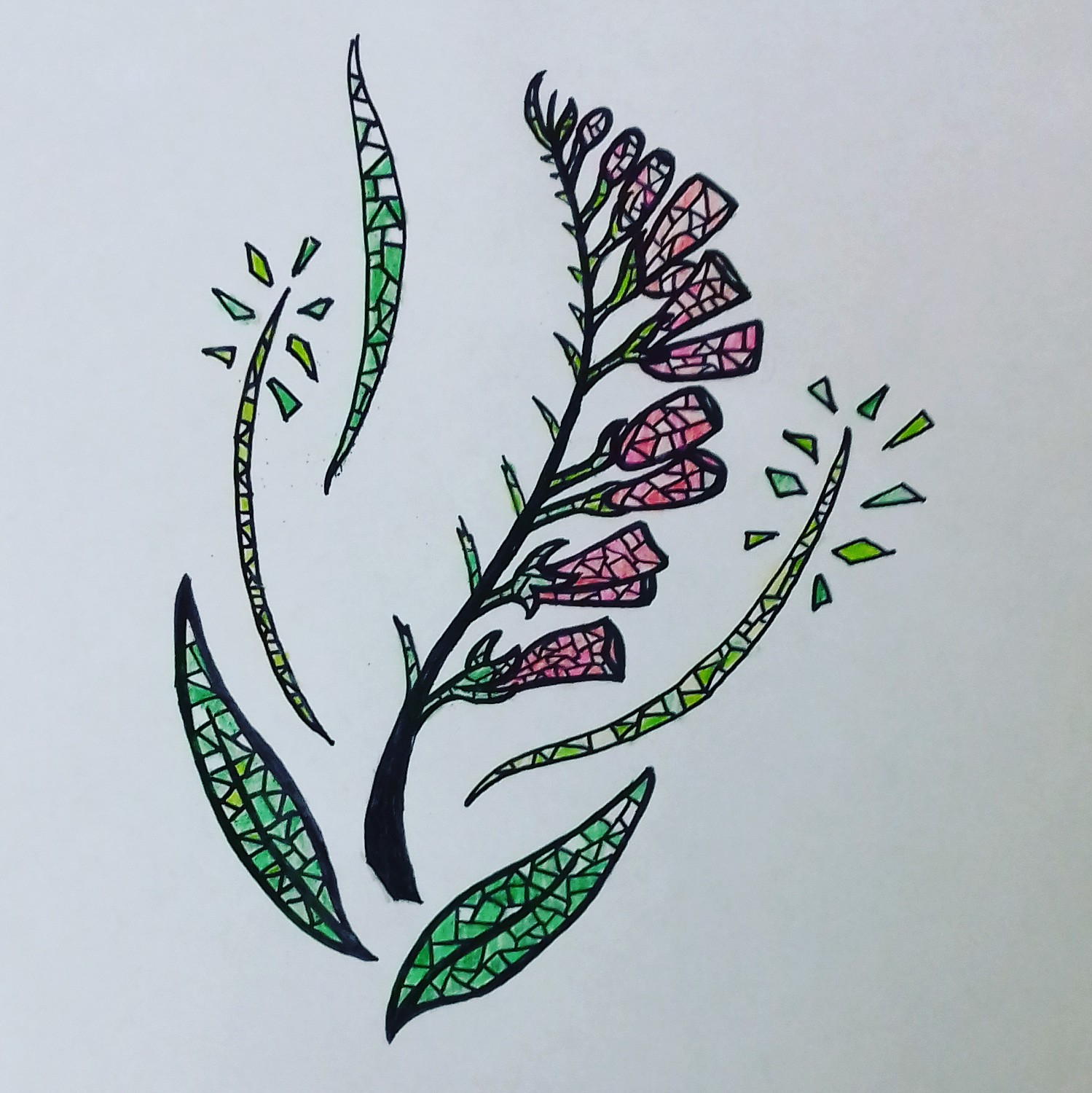This illustration features a botanical doodle, likely created with a black marker for the outlines and colored pencils for the vivid details. The central focus is a slender black branch that ascends from the bottom of the image, adorned with an array of more than a dozen pink floral bulbs emerging predominantly from its right side. Interspersed among the blooms are several unattached brown leaves, adding an extra layer of interest to the composition. Distinctly, the body of the flowers, leaves, and branch sections are segmented into geometric shapes such as triangles, squares, and rhombuses, resembling a mosaic pattern. The predominant color of these geometric sections is green, contrasting beautifully with the pink hues of the floral bulbs and the stark black of the branch, giving the entire piece a stained-glass window effect.